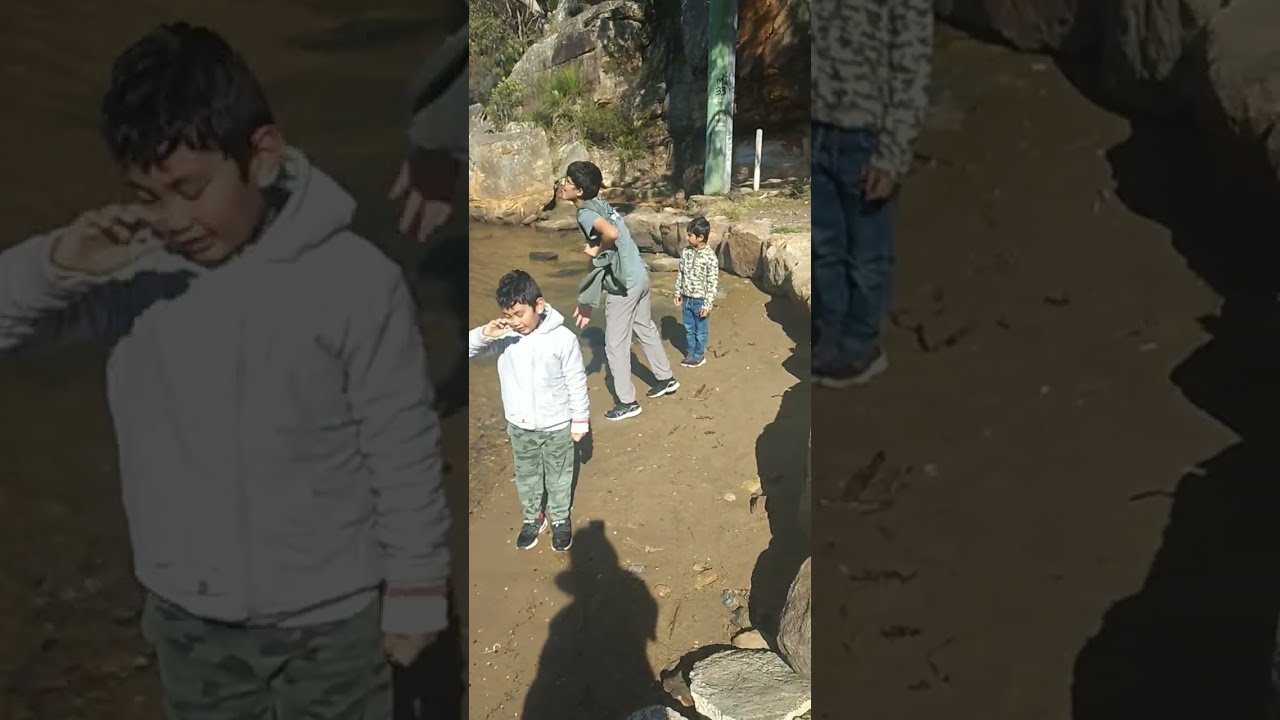This vertical, color photograph, likely taken on a cell phone, captures three prepubescent boys standing together in a circular, outdoor setting. The area is framed by large, gray rocks and has a brown, muddy ground, scattered with pebbles and stones. The boys, dressed in casual attire, are positioned in an environment that resembles a zoo or a natural area. They are surrounded by rocks, plants, and a wooden greenish pillar or tree. The setting is well-lit, indicating daytime, with plenty of natural light highlighting the scene.

The boy in the foreground on the left is dressed in a gray hooded sweatshirt and mottled green and brown pants, wearing black sneakers, and has one hand raised to his face, eyes closed as if wiping something away. Behind him, a taller boy appears to be interacting with someone out of frame. This boy wears a bright green t-shirt, gray pants, and black sneakers. The smallest boy, further in the background, sports a zip-up top with a camouflage pattern, blue jeans, and dark shoes. The overall terrain is accentuated by surrounding green plants and a large moss-covered rock, giving the scene a natural, earthy feel. In the bottom middle of the image, the shadow of the person taking the photograph is visible, adding a subtle sense of presence and perspective to the composition.